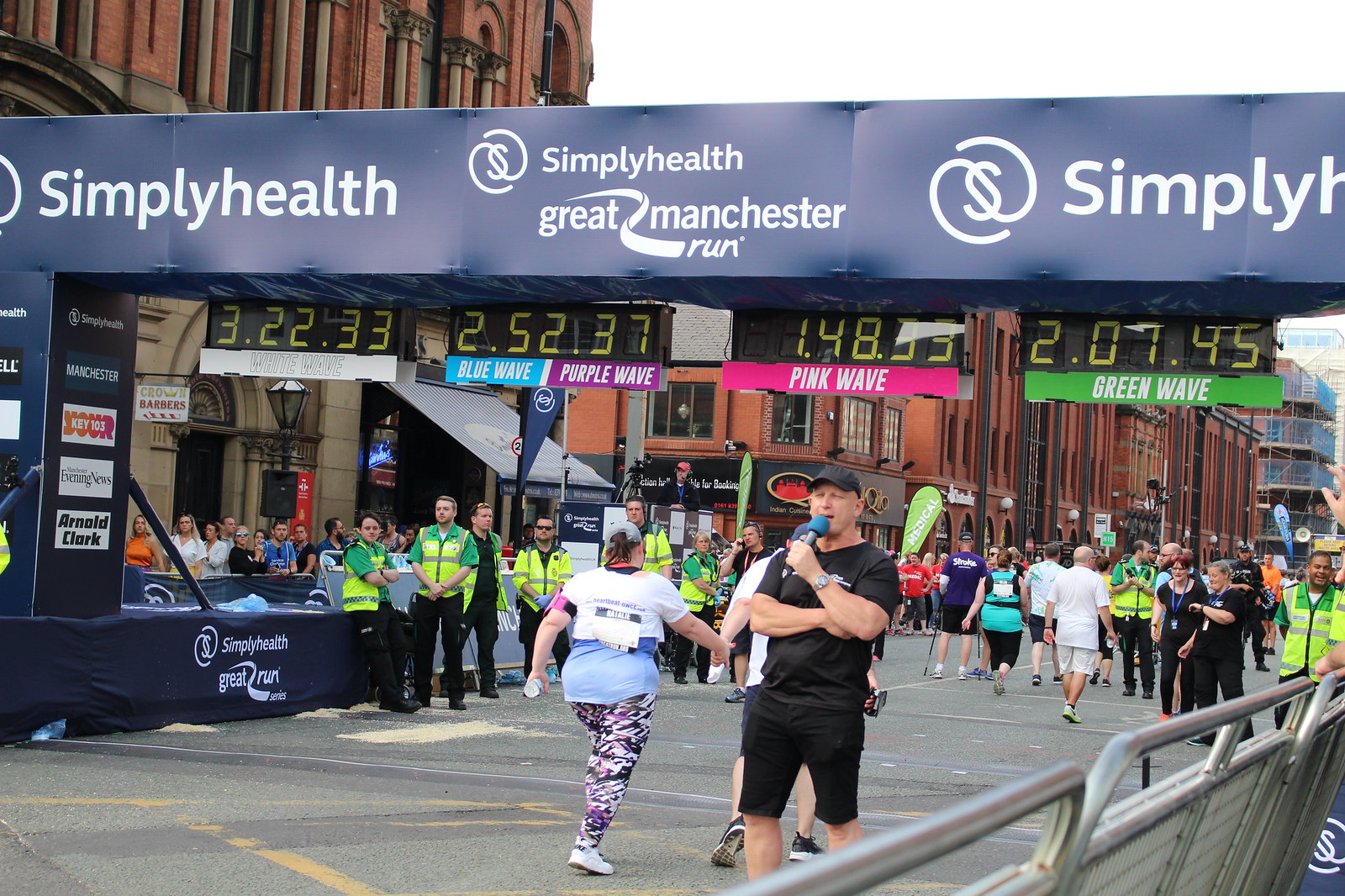This detailed photograph captures the bustling finish line of the Simply Health Great Manchester Run. Dominating the scene is a large makeshift archway adorned with advertisements, primarily showcasing the event's sponsor, Simply Health. Timers on the archway display finishing times for different waves: Pink wave at 1:48:53, Green wave at 2:07:45, Blue wave at 2:52:37, and White wave at 3:22:33. In the foreground, a man dressed in a black t-shirt, shorts, and cap holds a microphone, presumably announcing the arrival of runners. 

Participants, many of whom appear to be amateurs identifiable by their varied physiques and leisurely pace, steadily cross the finish line. They are equipped with race bibs and some wear green and yellow tops, possibly indicating affiliation with the event's organizers. On the left, a woman in athletic gear with a white race bib pinned to her back has just completed the race. There's also an emergency personnel presence, distinguishable by their vests. 

Cheerful spectators line the race route, held back by silver barricades on the right side. The backdrop features a mix of red brick buildings and structures typical of an urban environment, enhancing the communal and celebratory atmosphere of the event.